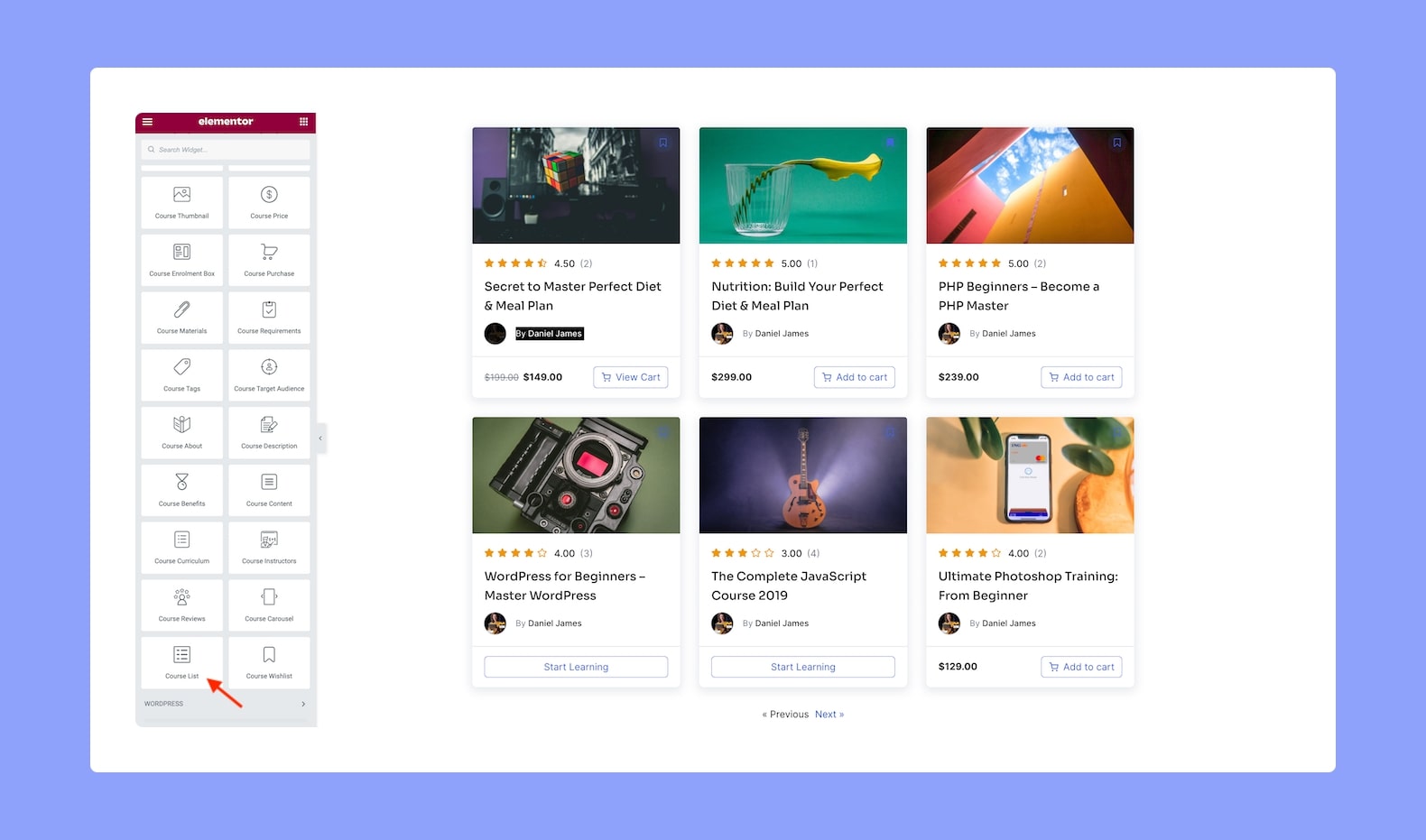This image is a detailed screenshot of a user interface featuring a complex layout. On the right-hand side, aligned towards the center, there are six distinct rectangular blocks. Adjacent to these blocks, running vertically from top to bottom on the left-hand side, is a menu. This menu is highlighted with a red bar at the top and includes a title. The menu is structured into two columns, encompassing a total of nine rows, thereby displaying two items per row.

Within the six blocks on the right:
- The top section includes three blocks:
  - The first block on the left is titled "Secret 2 Master Perfect Diet and Meal Plan," priced at $149.
  - The second block is labeled "Nutrition: Build Your Perfect Diet and Meal Plan," with a listed price of $200.
- The bottom section also consists of three blocks, among which:
  - The block on the bottom right is titled "Ultimate Photoshop Training for Beginners."

This comprehensive interface appears to be a well-organized informational or product display, meticulously categorizing items by their characteristics and prices.